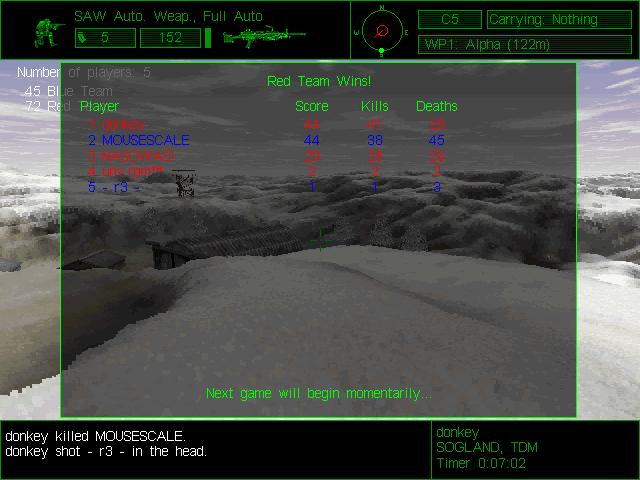This is a screen capture from a military-themed video game, depicting a pause or transition screen. The top portion features a black rectangle with a green banner displaying “SAW, AUTO, WEAPON, FULL, AUTO,” indicating weapon settings. Next to this, there's a directional compass for navigation. Below these elements, the center of the screen shows a gray overlay with columns listing players, scores, kills, and deaths, prominently displaying “RED TEAM WINS” signifying the end of a match. The player statistics include details like 72 red team kills versus 45 blue team kills and individual actions such as “DONKEY KILLED MOUSE SCALE” and “DONKEY SHOT R3 IN THE HEAD” with corresponding times. In the background, the rendered terrain resembles either snow-covered hills or a mountainous desert. At the bottom, white text reads, “Next game will begin momentarily,” indicating the pause before the next round begins. Additionally, an image of a crouching soldier in uniform is visible on the left side, enhancing the military atmosphere of the game.